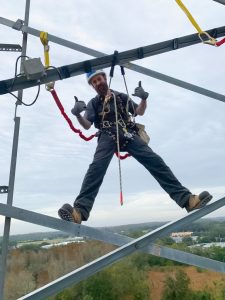In this grainy photograph, a construction worker is depicted high above the ground, balancing on a complex metal scaffolding structure. Dominating the frame, the worker's figure adds a sense of scale and height to the scene. He is positioned amidst an intricate network of grey metal beams, forming X-shaped cross supports both above and below him. Detailed straps secure him in place, with a prominent yellow strap and a red strap connecting his safety harness to the structure. 

The worker, who is the central focus of the image, sports dark blue overalls, a white hard hat featuring a blue rectangle on the front, and grey gloves. His relaxed stance, with legs apart and weight supported by the harness, conveys confidence and ease. He enthusiastically displays the shaka hand gesture with both hands, his grinning face framed by a thick brown beard. His rugged look is completed with brown work boots featuring black toes.

In the background at the base of the frame, a green and brown forest gives way to a collection of white and orange-ish brown buildings, indicating a small town rather than a bustling city. The sky above is filled with grey clouds, adding a muted tone to the scene. This atmospheric image, likely captured by a fellow worker, captures the camaraderie and high spirits of the crew despite the challenging and elevated workspace.